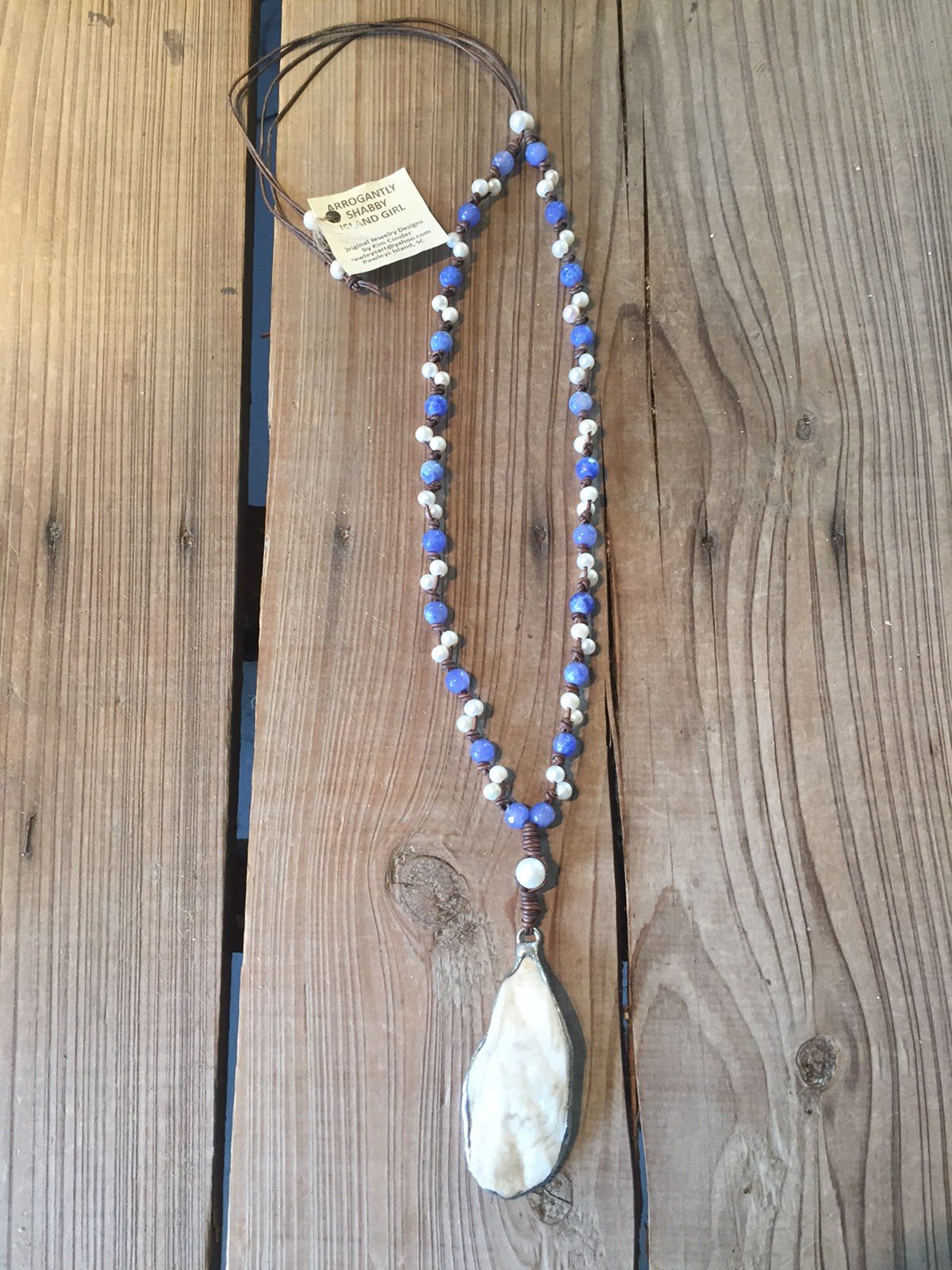The image showcases a handmade necklace placed on a rustic, barn wood background with three weathered boards featuring knots and a gray hue. The necklace, identified as "Arrogantly Shabby Island Girl," is intricately designed with blue and white beads strung along a black cord. It culminates in a pendant at the center, which appears to be a piece of white shell or rock wrapped with additional cord and fitted with a jump ring. The pendant also features a distinctive white bead in its center. Attached to the necklace is a tag displaying the brand name. The scene seems to be lit by natural sunlight, which casts a gentle glow across the setup, adding to its artisanal charm.